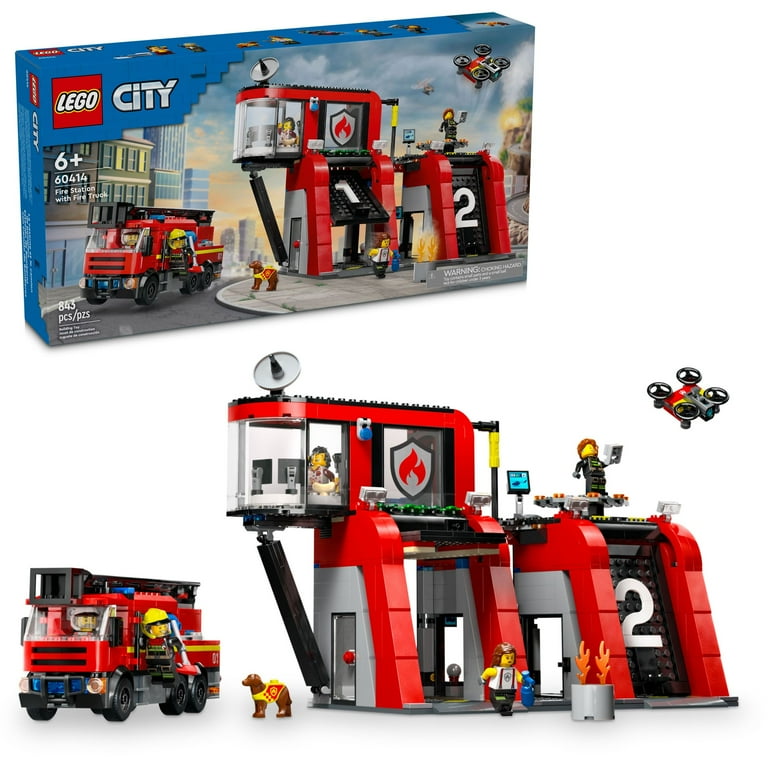The image showcases a LEGO City set, prominently featuring both its box cover and the fully assembled model beneath it. The box, at the top half of the image, highlights that this set contains 843 pieces and is suitable for builders aged six and up. It depicts a detailed, futuristic fire station scenario identical to the assembled set shown on the bottom half.

The completed LEGO set vividly demonstrates a modern fire station theme. On the left side, a red fire truck is depicted with two firefighters; one is driving, while the other clings to the door handle wielding an axe. Adjacent to them, a small brown dog dressed in a yellow and red fire vest stands alert.

The right side of the image features the fire station, characterized by its sleek, contemporary design. The top level houses a control center with expansive glass bay windows, inside of which sits a dispatcher monitoring two computer screens. Atop the station, a satellite dish enhances its high-tech appearance, while nearby, a firefighter operates a four-rotor drone equipped with a camera.

Below, another firefighter exits the building, seemingly heading towards a small fire, clutching a fire extinguisher. Every intricate detail in this LEGO set's assembly speaks to its complexity and the immersive play experience it offers.